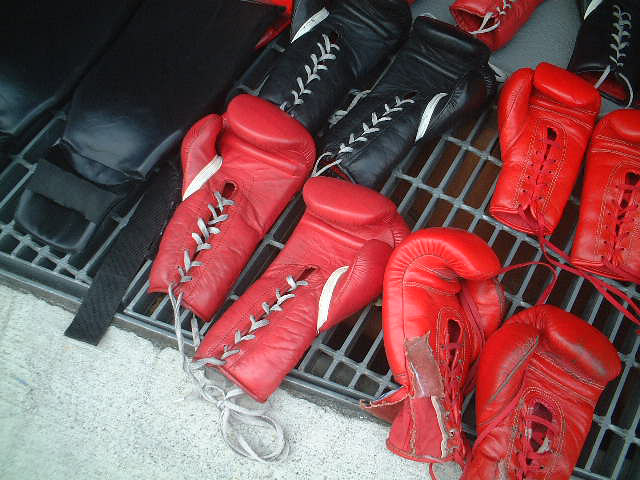This image is a detailed photograph taken from a bird's eye view displaying an assortment of boxing gloves laid out on a metal rack near the ground, revealing some of the concrete surface below. There are six pairs of boxing gloves visible in the image, comprising four red pairs and two black pairs. Three of the red pairs are prominently visible, with one partially cut off at the top. Similarly, of the black pairs, one is almost entirely in view while the other is partially cut off at the top. Each glove is equipped with characteristic white or red laces, intricately tied through holes that run from the thumb, around the palm, and down to the wrist. Some of the gloves show noticeable wear and tear, with one appearing quite old and another relatively new. Adjacent to the gloves lies an unidentifiable object resembling a rectangular piece of leather or a black padded fabric item. The metal rack they rest on has openings, suggesting it might cover a space below.